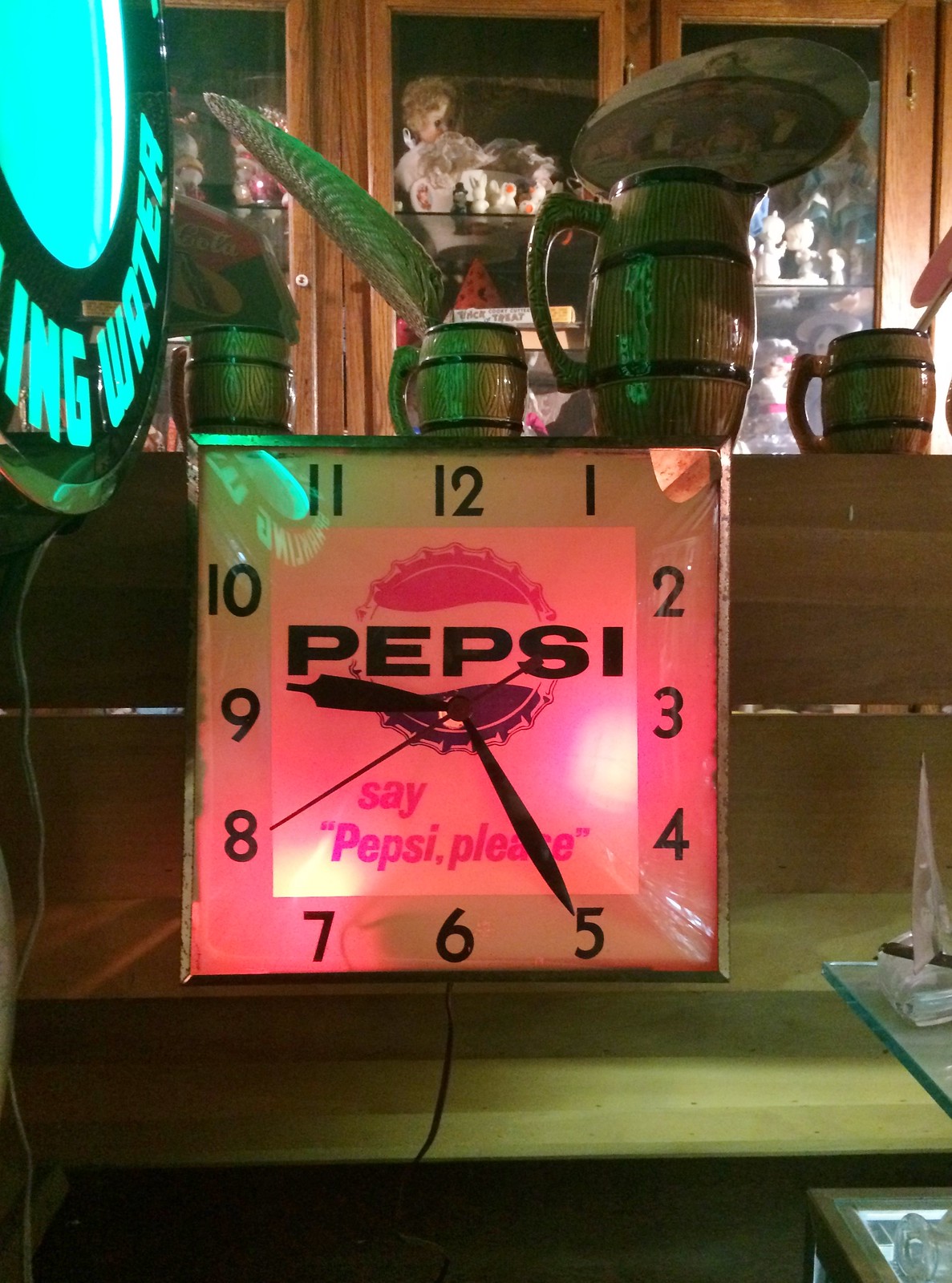This image appears to be set in a cozy, rustic bar. The centerpiece of the photograph is a vintage, square-shaped plastic clock, prominently displaying the time as 9:25. The clock is adorned with an old-fashioned Pepsi logo featuring the nostalgic red and black crown bottle cap design, and the phrase, "Say Pepsi, please," is emblazoned across its face. The clock's numbers are in standard American numerals from 1 to 12.

The clock rests on a sturdy wooden table, adding to the warm, vintage atmosphere of the bar. In the background, three ceramic tankards, reminiscent of traditional German beer mugs, are neatly lined up in front of a glass shelf. This shelf is filled with an eclectic collection of decorative items, contributing to the bar's charm and character. The entire scene evokes a sense of nostalgia and timelessness, capturing a moment in a quaint, inviting setting.